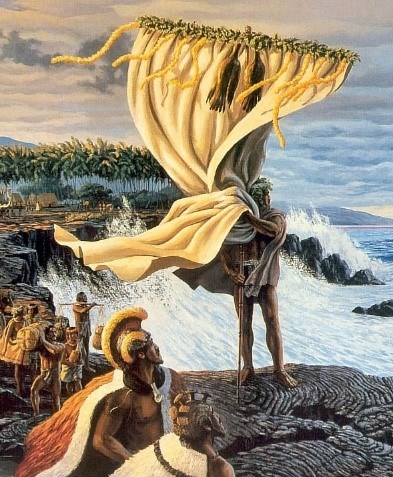In this detailed illustration evoking ancient times, potentially set in ancient Rome, a tumultuous coastal scene unfolds with waves violently crashing against a rocky shoreline shaped in a semi-circle. Central to the image is a man, possibly a Roman gladiator, standing resolutely on the rocky shore. He holds a tall staff adorned with a white cloth draped down, fluttering like a banner. His cloak billows behind him, and his presence commands attention from two other nearby gladiators, both looking up towards him. These men wear armored headgear and are shirtless but draped in capes, with their muscular forms meticulously depicted by the artist.  

In the background, a group of individuals, perhaps depicted as Indigenous persons mourning or engaging in labor, can be seen carrying various goods and baskets on sticks across their shoulders. They are shirtless as well, wearing fur stoles or mourning clothes, emphasizing their varying cultural attire. Stylized palm trees wave in the distance, adding a tropical detail to the otherwise dark and stormy day. The scene’s rich color palette includes shades of brown, gold, red, white, and blue, contributing to the dramatic and realistic mood of the artwork. No text or labels are present in the image, allowing the visual elements to tell the story of this intense moment on the storm-battered shore.